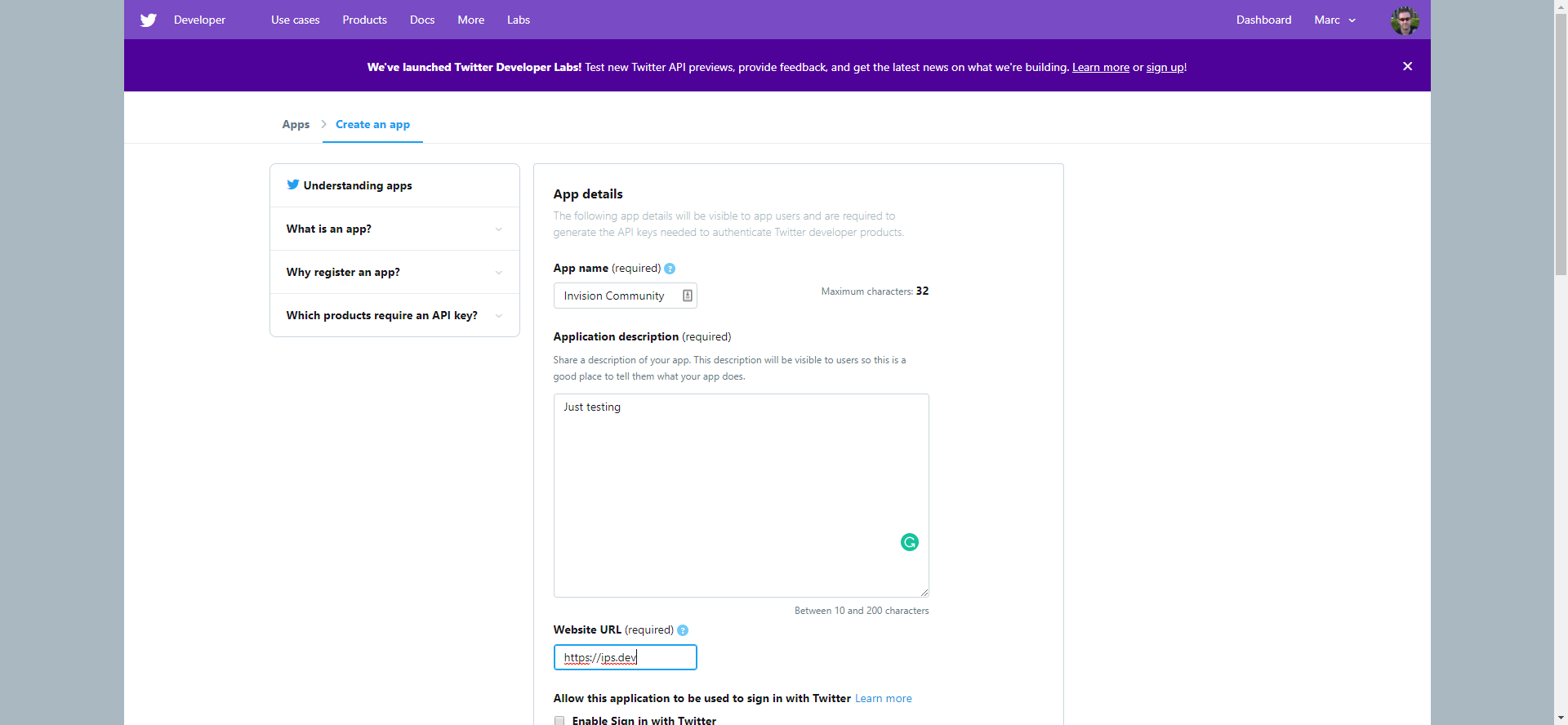A panoramic, rectangular image showcases a highly detailed interface, presumably of a web development tool. At the very top of the picture, a light purple bar stretches the entire width, featuring a white "XBird" logo on the left, resembling the new Twitter logo. To the right of the logo, white text that reads "Developer" is followed by unclear, smaller words. Further right, the readable sections include "Podcast," "Docs," "More," "Less," and "Dashboard." The upper right corner prominently displays a white downward-facing triangle. Adjacent is a small circle with a tiny avatar, possibly depicting a Caucasian male, though it’s difficult to discern.

Below the header is a darker purple bar with white text. The legible portion reads, "We've balanced Twitter designer label," ending with "Learn more," which is hyperlinked. A white 'X' icon appears to the right of this bar.

The main content area is dominated by a large white space. In the upper left, the word "Apps" in black is accompanied by a right-facing gray triangle and aqua blue text "Create an App," underlined with the same aqua hue. Below "Apps," a gray line separates the large white area, revealing a white box containing clickable options: 

1. "Understanding Apps" with the blue Twitter bird icon.
2. "What is an App?"
3. "Why register an app?"
4. "Which products require an app API?"

A faint gray-rimmed box follows, with text too small to read clearly. The top-left corner reads "App Details" in black. Below, to the left, "App Name (required)" is indicated with a blue circle. A text box displays partially readable content, including the word "community." Alongside the box, black digits "32" are paired with phrasing that's challenging to make out.

Beneath, another section labeled "Application Description (required)" appears, followed by a large white, gray-rimmed box for inputting details. This box has "Just testing" written in black at the top left and a Gmail logo towards the lower right. Just outside and below this box, a character count feature is faintly visible.

The final segment on the left displays "Website URL (required)" with a blue circle next to it and another text box below. This box contains text with red misspelling bars underlined. Finally, at the bottom, black text—too small to read—ends with blue hyperlinked text that likely says "Learn more."